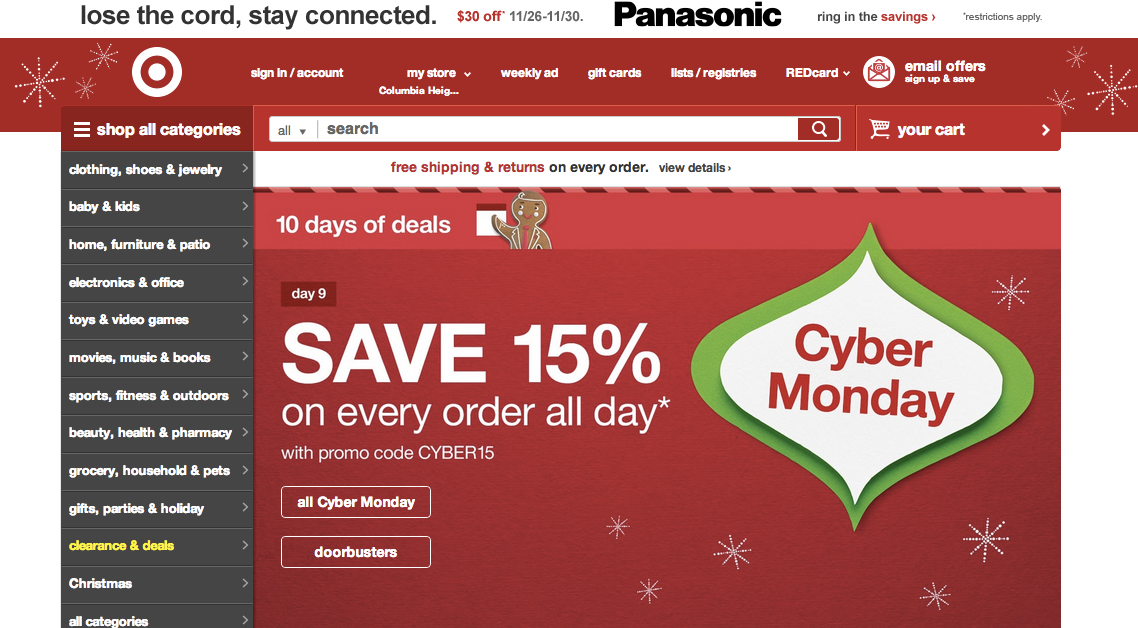The image features a solid white background with red and black text elements arranged in a promotional format. At the top, there's a prominent red rectangle hosting a bold black text that reads: 

"Lose the cord; stay connected. $30 off 11/26 through 11/30 on Panasonic. Ring in the savings. Restrictions apply."

Beneath this, there is a red banner displaying the iconic Target logo on the right side, accompanied by navigation options such as "Sign In," "Account," "My Store: Columbia Heights," "Weekly Ad," "Gift Cards," "Lists," "Registries," "RedCard," and "Email Offers."

Dominating the middle section of the image is a larger red banner with a compelling message in big white text:

"Save 15% on every order all day with promo code CYBER15."

Underneath this message, two smaller white outlined boxes are noted, reading "Cyber Monday" and "Next Door Busters". 

Along the left edge of the image, positioned vertically, is a list of shopping categories in white text against a black background. These categories include:

- Clothing, Shoes & Jewelry
- Baby & Kids
- Toys & Video Games
- Beauty
- Health & Pharmacy
- Gifts, Parties & Holiday